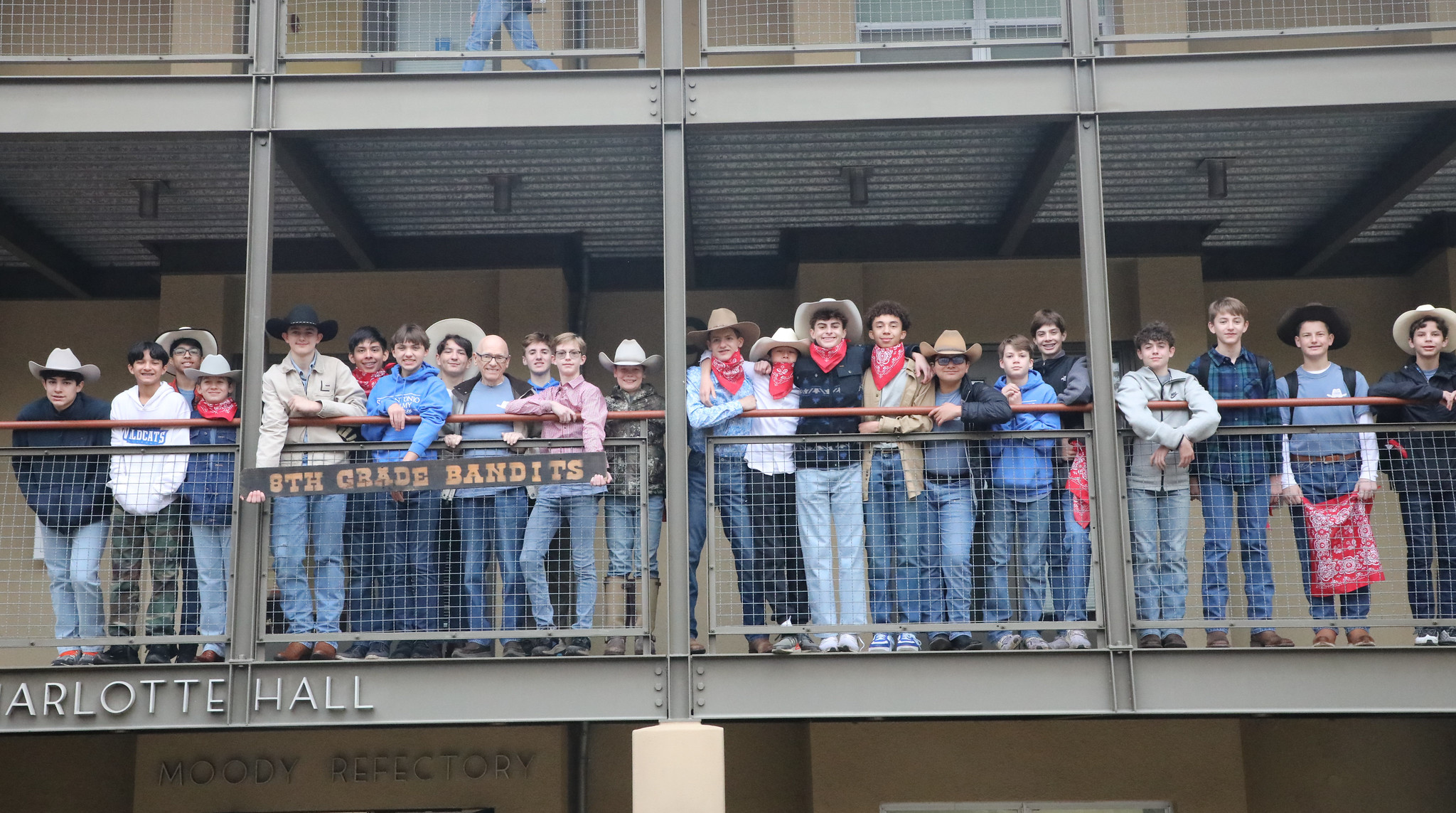In this vibrant photo, a group of boys, predominantly 13 or 14 years old and dressed in country attire, stands on a second-story deck against a mesh metal railing. The boys, mostly clad in blue jeans and jackets, are adorned with red and white bandanas around their necks or in their hands, and many sport cowboy hats in various shades of white, black, and beige. They are beaming with smiles as they hold up a large wooden plaque about 6 feet long that reads "8th Grade Bandits" in beige lettering on a gray background. Also visible in the scene are the names "Charlotte Hall" and "Moody Refectory" on the building behind them, suggesting a school setting. At least one older male, likely their teacher or chaperone, is also present, enhancing the sense of camaraderie and celebration among the group.